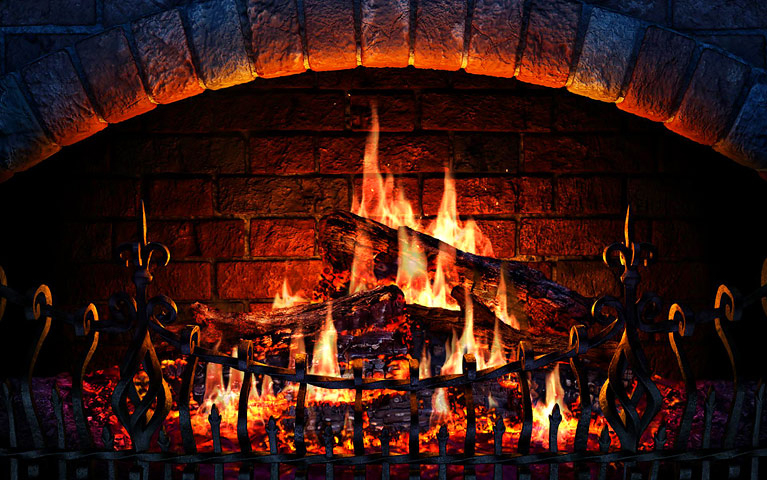In the image, we see a detailed close-up of a fireplace illuminated solely by the flames within. The background reveals the red brick structure of the fireplace, with the top arcs of bricks stretching from the left and rising toward the middle before descending slightly on the right, partially shadowed but tinted orange by the fire's glow. Dominating the foreground is a black iron gate stretching horizontally across the scene. Behind the gate, there are three logs stacked atop each other, their surfaces blackened and accented with hints of blue from the heat. The roaring fire emanates vibrant hues of orange, white, and red from these logs. Below the grate, through its intricate design, you can spot glowing coals in shades of black, orange, and yellow. The overall scene is a vivid depiction of a crackling fire, capturing both the serene and intense aspects of the flames in the cozy hearth.